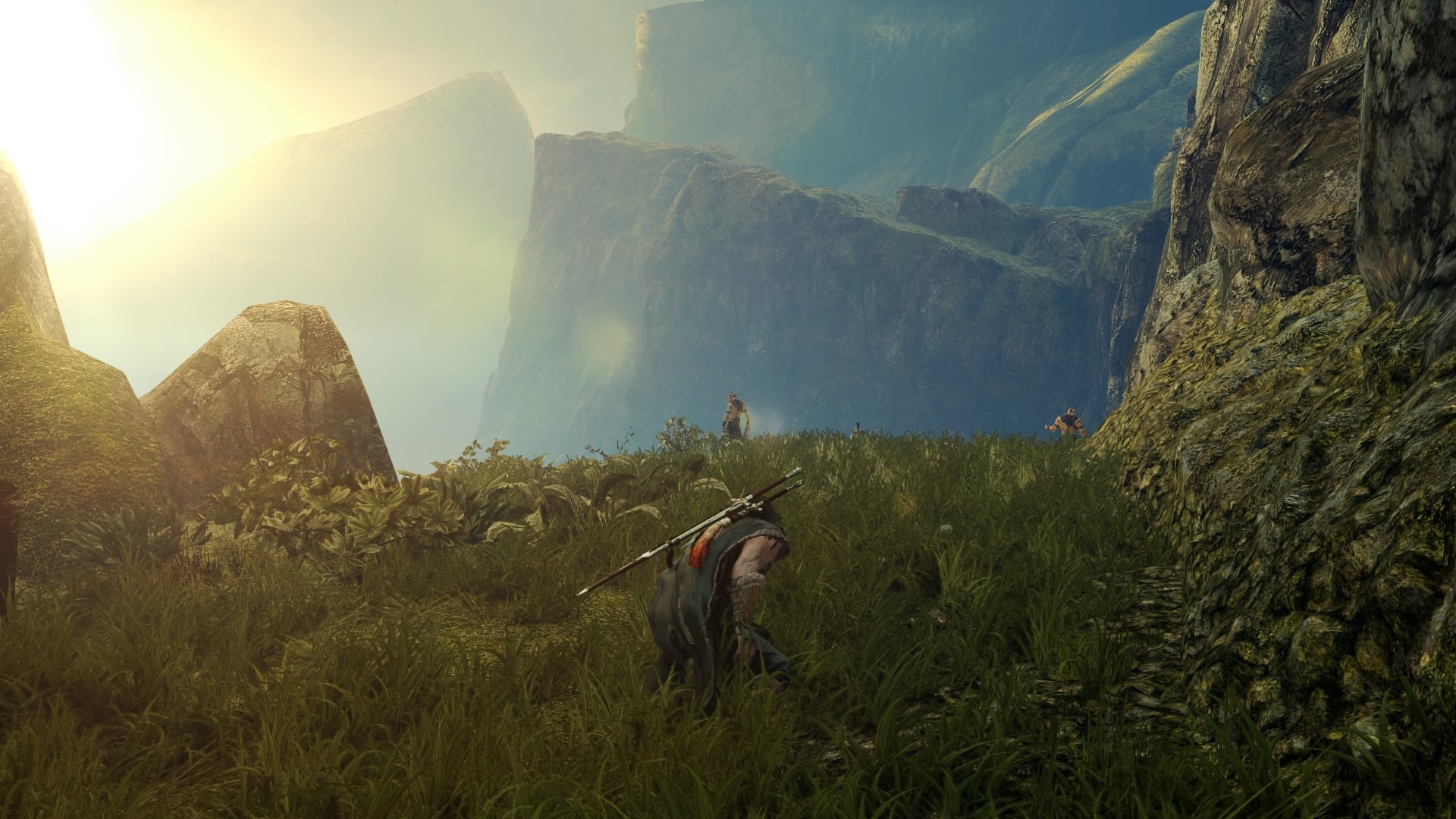The image depicts a highly detailed, computer-generated art print of a mountainous landscape, dominated by sharp vertical cliffs with angular edges. In the foreground, a tribal-like warrior, attired in a taupe long-sleeve shirt and a black cape-like garment, is crouched over in tall, wild grass. This warrior has a long silver sword with a black handle and a shorter sword on his back, accompanied by a conspicuous white and orange feather. The grass is depicted in a medium green hue, adding a natural vibrancy to the scene. Surrounding the warrior are vivid wildflowers dotting the ground. To the right, a steep vertical cliff face rises dramatically, while in the middle distance, two tiny figures are seen on the edge of what appears to be another cliff, their exact activity unclear. The background reveals a series of hazy, gray and brown mountainscapes with some moss covering, fading into lighter areas under the diffuse glow of a hazy sun in the upper left. A distinct arch carved into one of the mountains on the right adds to the rugged terrain's mystique. The overall atmosphere is imbued with a surreal, video game-like quality, emphasizing the grandeur and isolation of nature, as the warrior seems to be engaged in a quest or search amidst the imposing scenery.